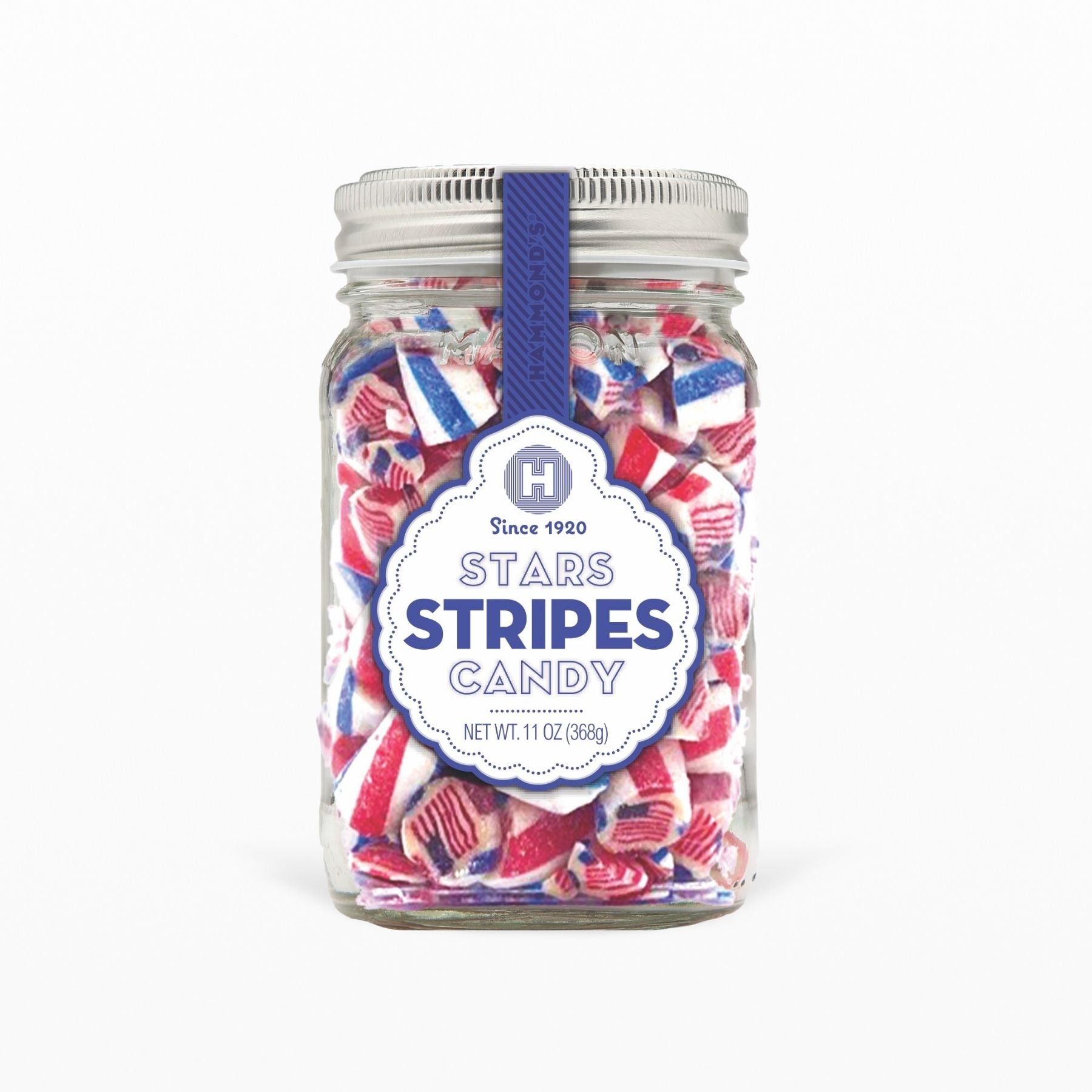This is a photograph of a glass jar with a metal screw-top lid, filled to the brim with hard candy colored in red, white, and blue. The candies inside resemble the American flag, sporting various stripes and stars. The jar is set against a grayish-white background, emphasizing its contents and label. The jar itself has a square form with a round, silver cap. A blue ribbon extends from the cap down to the center of the jar, leading to a blue circular label. The label features an "H" at the top and details such as "Since 1920" and "Stars, Stripes, Candy," along with the net weight of 11 ounces (386 grams). The photograph is clear and well-composed, likely intended for a product listing or promotional material.